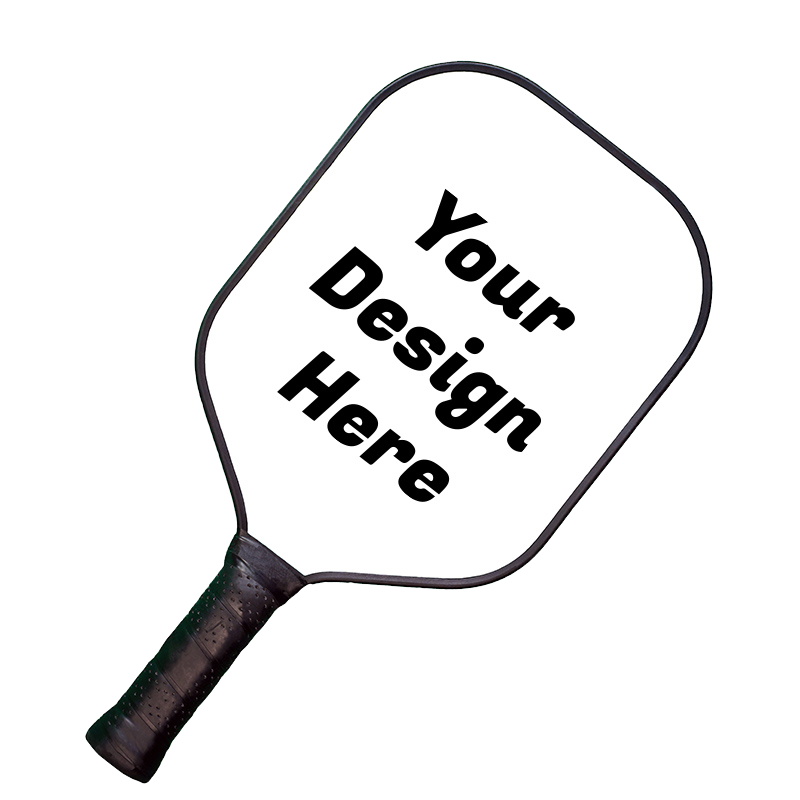The image depicts a solitary pickleball paddle placed sideways against a plain white background, giving it a floating appearance typical of product presentations on e-commerce websites. The paddle's handle is wrapped in black tape with small perforations for grip, implying practical use. The paddle itself features a black outline, adding a striking contrast against the white interior. In the center of the paddle, in bold, capitalized black text, it reads "YOUR DESIGN HERE," indicating customizable options for personal logos or designs.